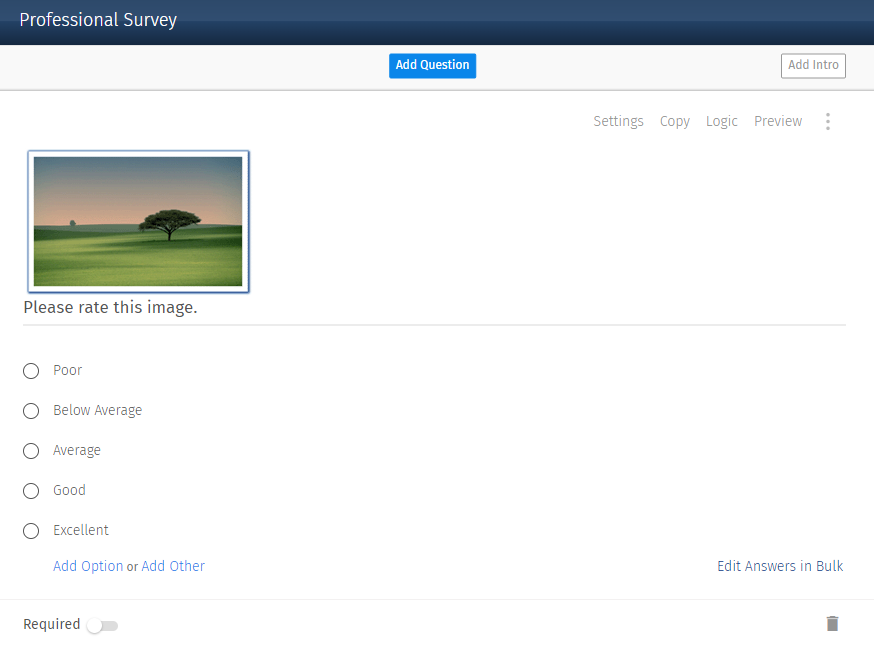The screenshot captures a webpage design meant for creating or editing a professional survey. The page has a dark banner running across the top, with the text "Professional Survey" prominently displayed in white on the left. Beneath this, a gray banner of the same width houses two buttons. In the center of the gray banner is a blue rectangular button labeled "Add Question" in white text, while on the far right is a white rectangular button labeled "Add Intro."

Below the gray banner, a thin gray line separates the header from the main content area. The main section is predominantly white and extends about a third of the way down the page. On the left side of this section, there is an image depicting a grassland with a single tree and a somewhat unrealistic, setting-sun skyline. Directly beneath the image, there is a prompt that reads, "Please rate this image."

To the right of the image, several interface elements are laid out in light gray text. These include options for "Settings," "Copy," "Logic," "Preview," and a three-dot menu for additional options. Below these, another thin gray line divides this area from the rating section.

The rating section features a vertical list of five options—Poor, Below Average, Average, Good, and Excellent—each accompanied by a radio button for user selection. Below this list are two clickable links in blue: "Add Option" and "Add Other." To the left of these links, there is another interactive link, "Edit Answers in Bulk," also in blue.

The final section includes a "Required" toggle button on the left, which can be adjusted by dragging a circle to the right or left. At the far right of this section is a trash can icon for deleting the question or section.